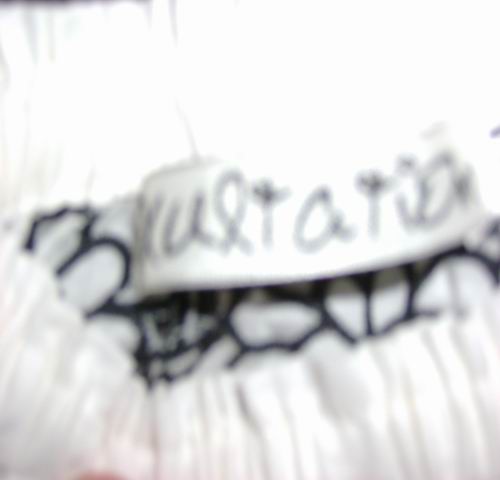This is an excessively blurry and low-resolution photograph, making it difficult to discern specific details. The image predominantly features a white cloth item that appears bunched up at the front edge, likely due to an elastic band or drawstring. A strip of writing is present in the middle of the image on a band similar to what might be found on the inside of underwear or a hat, though the text is too unclear to decipher fully. The most recognizable letters might suggest "K-U-L-T-A-T-O" but this is speculative. The white background is blown out by highlights, resulting in a lack of visible detail in those areas. Additionally, there is a black and white floral or line art pattern that extends across the cloth item. A red object is vaguely discernible at the bottom left, but its exact nature cannot be determined. The photograph suffers from significant blur and poor quality, with bright white areas overpowering other details, further complicating identification of the item.